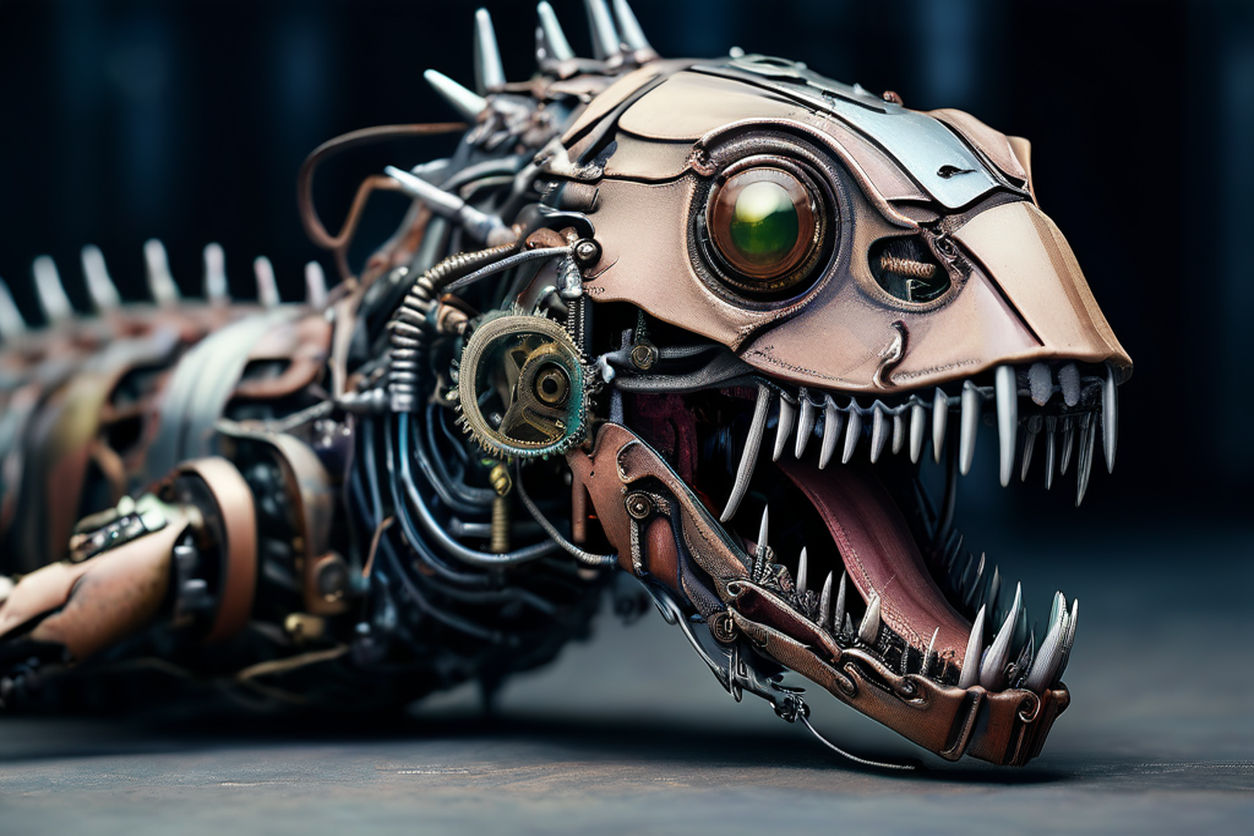This photograph captures a highly detailed, mechanical creature resembling a dinosaur or some sort of fantastical lizard. Dominating the composition is a close-up of the creature's head, slightly right of center. The head appears to be constructed from various pieces of scrap metal and brown leather straps, all patched together to form a coherent yet complex visage. Its most striking feature is a large, camera-lens-like eye with a green pupil and a brown iris. Just below the eye is a nose hole.

The creature's mouth is open, displaying a set of long, narrow, metallic teeth that glint in the light, complemented by a rose-colored tongue that appears to be made of leather. The jaw itself seems crafted from leather with mechanical components protruding from the underside, connecting to the body via an intricate network of wires.

Moving to the body, which becomes progressively more out of focus, we notice it's chiefly composed of bronze-colored metal. The mechanical insides are visible through gaps, showing wires and gears reminiscent of a watch's inner workings. Along its spine, silver spikes jut out, giving it a menacing appearance. An appendage, possibly a flipper or an arm, extends off-screen to the left, making it difficult to ascertain its exact nature. 

The scene is set against a blue background with the creature resting on a gray surface, enhancing the detailed mechanical aesthetic and creating a stark contrast with the more organic elements of its design.